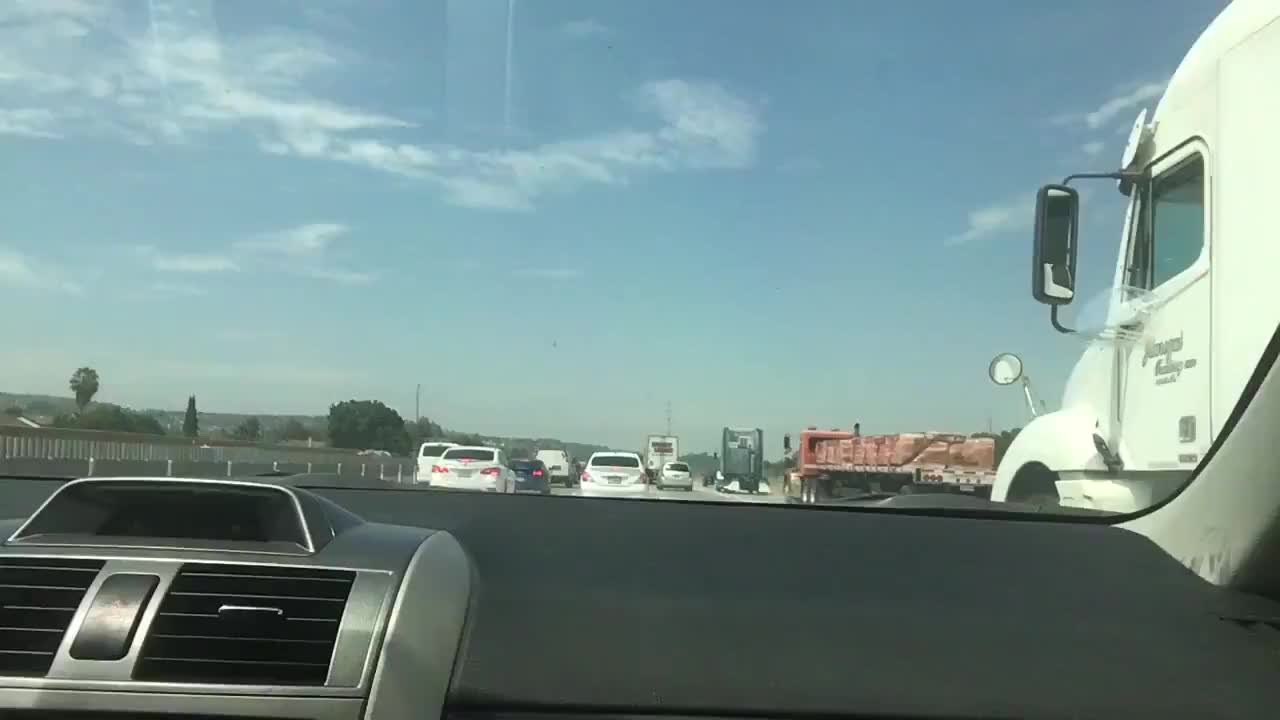This crystal-clear daytime photograph captures the busy scene from within a vehicle caught in heavy traffic. The image features a black dashboard with a silver center console and black air vents prominently visible. Through the windshield, a blue sky dotted with wispy white clouds creates a serene backdrop. Adjacent to the vehicle, a white truck with a prominent black side mirror is visible. In front of this truck, a red truck with a red-brown payload continues the line of traffic.

Directly ahead, a white sedan occupies the lane, while the opposite lane is populated by a darker-colored sedan and another white sedan. Further along, a pair of white vans can be seen, along with a distant silver minivan and another white truck. In the background, green trees offer a touch of nature amid the urban environment, while power lines and a guardrail further frame the congested roadway.